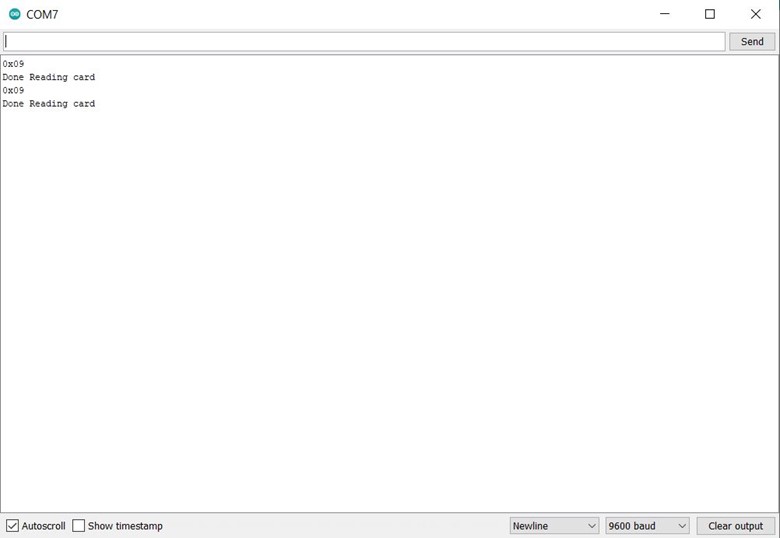The image displays a plain interface dominated by a window showing lines of code, likely from an Arduino Integrated Development Environment (IDE) designed for hobbyist electronics. At the top of the window, "COM7" is prominently displayed, signifying the active communication port. To its side, the distinctive Arduino logo is visible. The interface features a white background with an input field at the top for entering commands or code. Below this, there are four lines of text, including repeated phrases such as "0x09, done reading card," and "copied," which are likely status messages indicating that a card reading operation has been completed successfully. "0x09" suggests a hexadecimal value, although its specific context remains unclear. The bottom section of the window includes several control options for adjusting text editor settings like "autoscroll," "new line," and "baud," the latter referring to the data transmission rate.